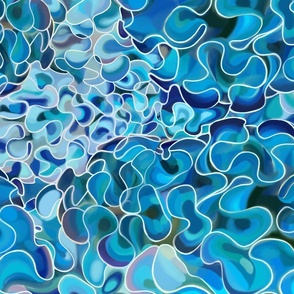In this abstract digital artwork, we observe a complex and detailed square image dominated by various shades of blue, from nearly white with a hint of blue to deep navy. The image is characterized by intricate swirls and squiggles, reminiscent of folds in a rosebud or puffy, irregular shapes akin to abstract letters. These elements are densely packed together, creating a visually busy and dynamic composition that evokes a sense of swirling, dizzying movement. Some sections are darker, while others feature concentrated, smaller spirals in lighter blues, with hints of greenish tints adding nuance to the palette. This multifaceted piece, resembling patterns one might find in a coral reef or reminiscent of jigsaw puzzle pieces, explores the chaotic beauty of abstract forms and colors.